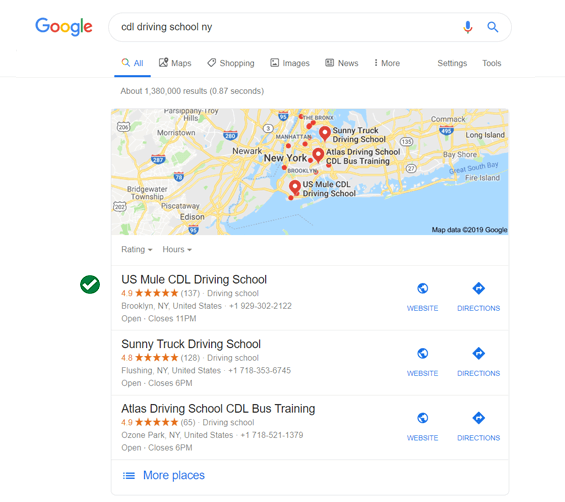The image depicts a Google search results page. The iconic Google logo exhibits its classic multicolored letters—blue, red, yellow-orange, blue, green, and red. Typed into the search bar is "CDEL driving school NY," and Google provides approximately 1,380,000 results in an impressive 0.87 seconds. 

Highlighted search results include "U.S. Mule CDEL Driving School," "Sunny Truck Driving School," and "Atlas Driving School CDEL Plus Training." Each result offers a link to the website and directions to the physical location of the driving schools.

Additionally, a detailed map of New York City is prominently displayed, showing various boroughs and landmarks. Notable areas such as Manhattan, Brooklyn, the Bronx, and Long Island's Bayshore are clearly marked. Locations of the search results are pinpointed on this map, indicating their proximity within the bustling metropolis.